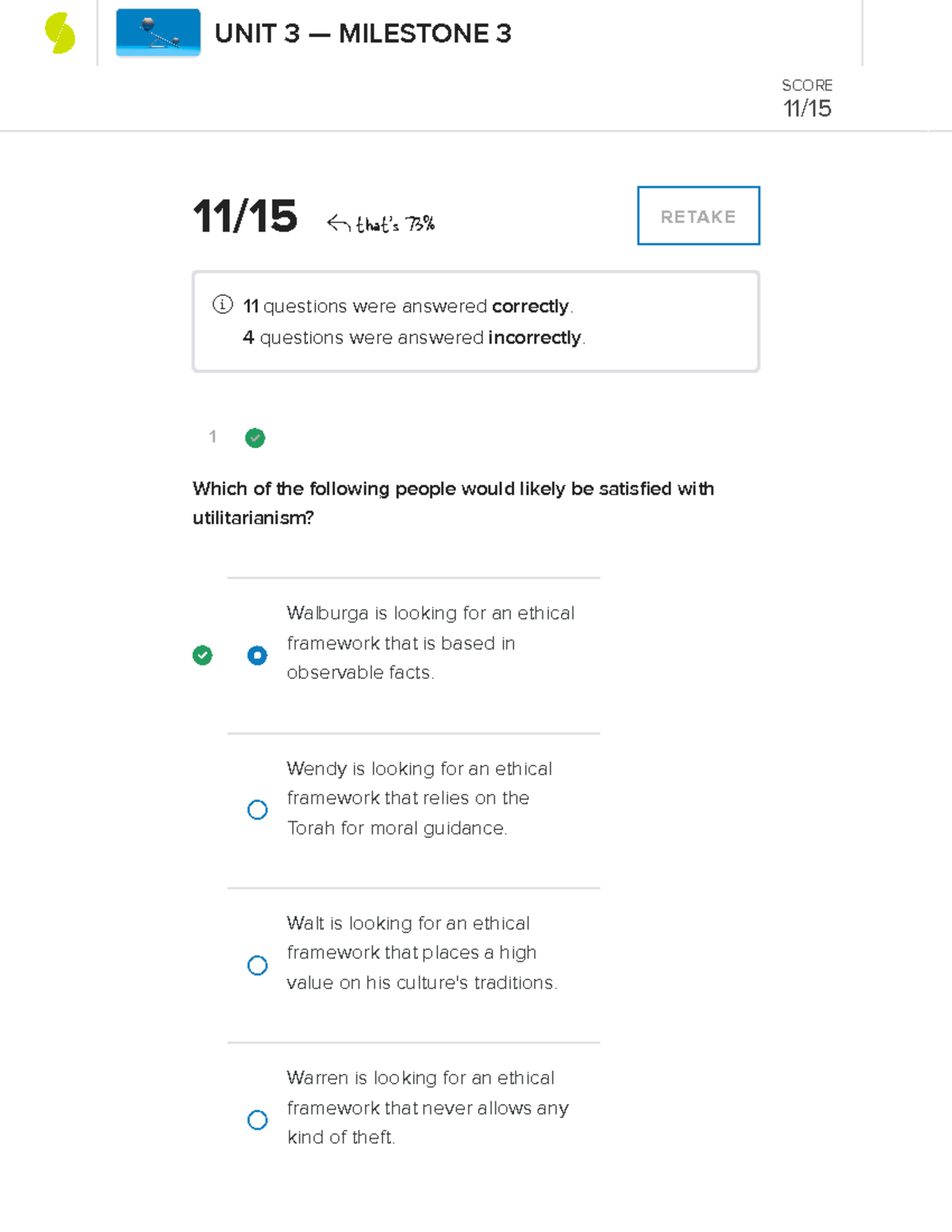This is a screenshot from Unit 3, Milestone 3, displaying the user's performance summary. The user achieved a score of 11 out of 15, resulting in a 73% accuracy rate. The interface prominently features a "RETAKE" option in a thin-lined blue box, encouraging attempts to improve the score. Additionally, details about individual questions are provided. For instance, the first question asks, "Which of the following people would likely be satisfied with utilitarianism?" The user chose the option, "Walburga is looking for an ethical framework that is based on observable facts," which is marked correct with a green tick. A grey box at the top of the screen indicates that 11 questions were answered correctly and 4 incorrectly. The overall design utilizes a black font for the main content, ensuring readability and focus.